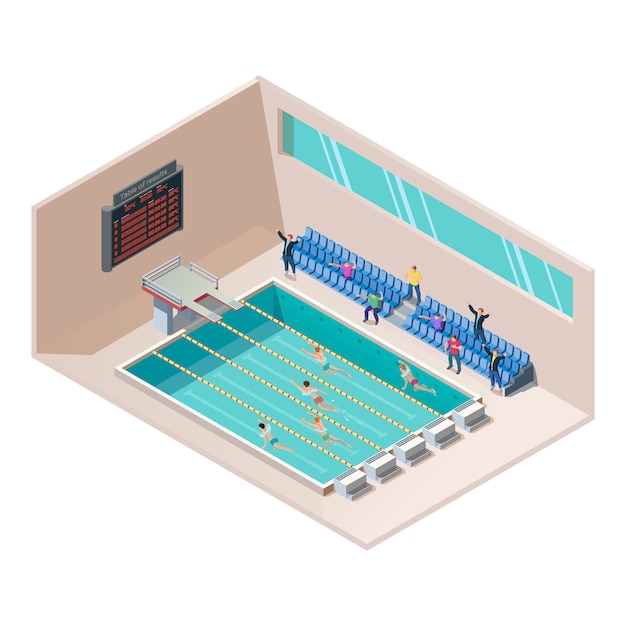The image is a detailed digital illustration of a competitive swimming scene, characterized by a clear yet stylized, unrealistic rendering. It portrays a five-person lap pool race, similar to what you might find in a corporate presentation or illustrative article about swim meets. Each swimmer is in a distinct lane, separated by yellow buoy ropes, swimming towards the left side of the image, where a diving platform with two diving boards is situated. The pool's water is a vivid blue, accented with white. On the far wall hangs a gray-bordered scoreboard with a black background and reddish-orange text displaying the title "Table of Results," indicating the swimmers' names and times. This scene is observed by a small, animated crowd of eight people in three rows of bleachers, enthusiastically cheering, some even performing "dab" poses. The swimmers, all depicted as male and wearing different colored swim trunks, are at various stages of the race, enhancing the dynamic and engaging nature of the illustration.